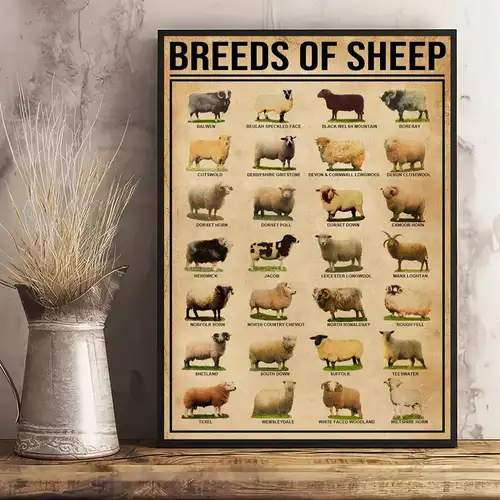On the left side of a rustic wooden shelf sits a silver tin vase, gracefully filled with an arrangement of long, beige and white grasses. The backdrop features a concrete-textured wall, adding an industrial touch to the setting. Hung prominently on the wall is an educational print titled "Breeds of Sheep," presented in bold black text. The poster meticulously categorizes various sheep breeds, organized into four rows. Each row displays a clear image of the respective sheep with its name labeled underneath, offering a visually engaging and informative element to the decor.